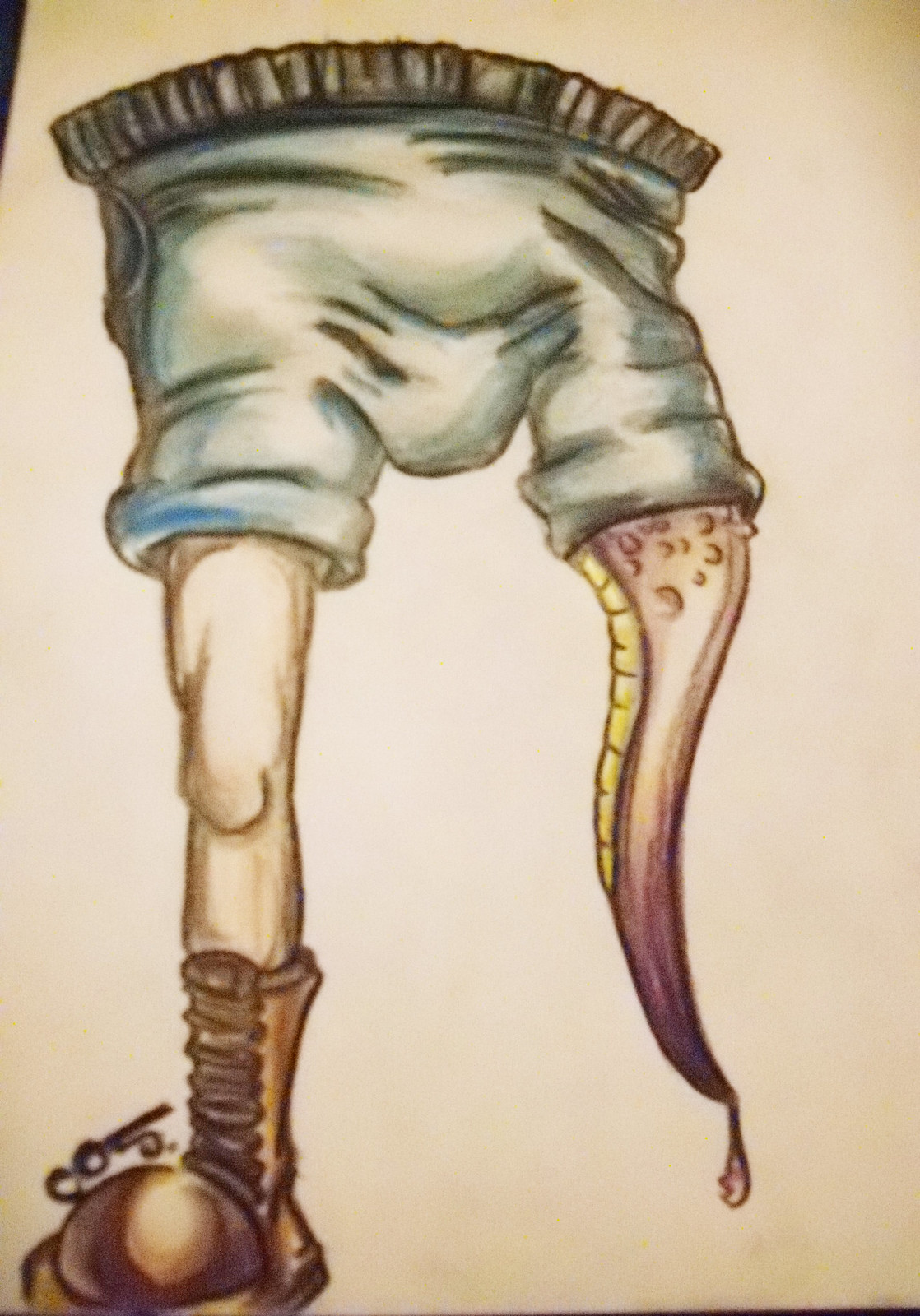This whimsical colored pencil drawing features the lower half of a man, rendered in a cartoonish style. The figure, from the waist down, wears what appears to be boxing shorts, which are wrinkled and scrunched, creating a saggy crotch area. Notably, the shorts have a distinctive black band at the waistband. The man's left leg (or the viewer's right) is muscular and clad in a heavy, brown work boot. In stark contrast, the figure's opposite limb is an octopus-like tentacle, extending downward from the shorts. The surreal combination of a human leg with a boot and an octopus tentacle contributes to the drawing's fantastical and quirky nature.